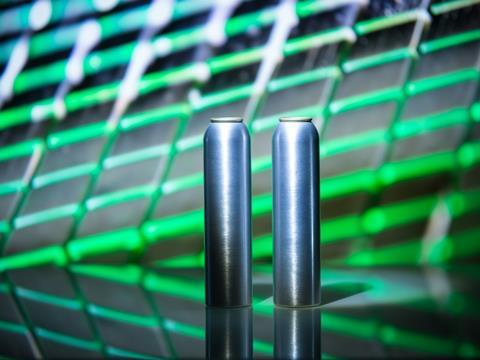The photograph features two reflective, silver metal cylinders standing upright on a highly polished, reflective metal surface. Each cylinder is capped with a slightly smaller disc, reminiscent of coins, giving the tops a rounded and tapered appearance. The reflective surface beneath them mirrors their form, as well as the netting and any light, casting discernible shadows behind the cylinders. In the backdrop, a blurry, neon green net made of metal stretches horizontally and appears slightly trapezoidal due to its angle. The background beyond the net is an indistinct, gray blur.